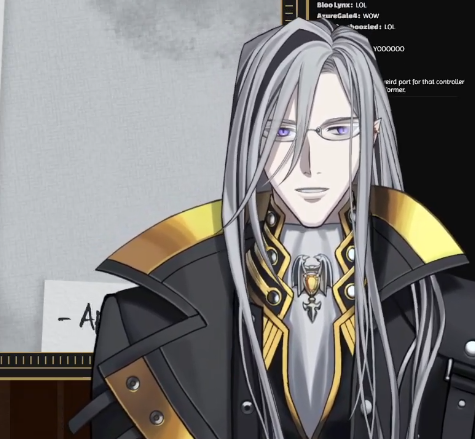The image features an anime-style character, a man likely in his twenties or thirties, with distinct long gray hair, sharp chin, and violet-purple eyes. He is wearing thin glasses and a black and gold jacket, resembling a trench coat or a heavy biker jacket, with a highly detailed popped collar edged in gold and adorned with gold buttons. Underneath, he is dressed in a gray shirt featuring an eagle emblem with a gold gemstone at its center. Notably, his face has a pasty white complexion indicating possibly a vampire or elf origin due to his pointed ears.

In the background, there are two boards visible: a blackboard and a whiteboard. The blackboard, located behind most of his head and left shoulder, contains typed text that reads “LOL, WOW, OK, OO,” among other indistinct messages appearing as if people are texting back and forth. To the left, there's a grayish-whiteboard with a ruler-esque black and gold border. Partially hidden by the man's jacket, there’s a piece of white paper on this board featuring a dash and an 'A' in black ink.

Behind and to the bottom right, there's a gray wall with a black shelf that holds another piece of white paper, again displaying a dash and an 'A.' The setting appears to be some kind of academic or office space, adding context to the character's scholarly or intellectual appearance.